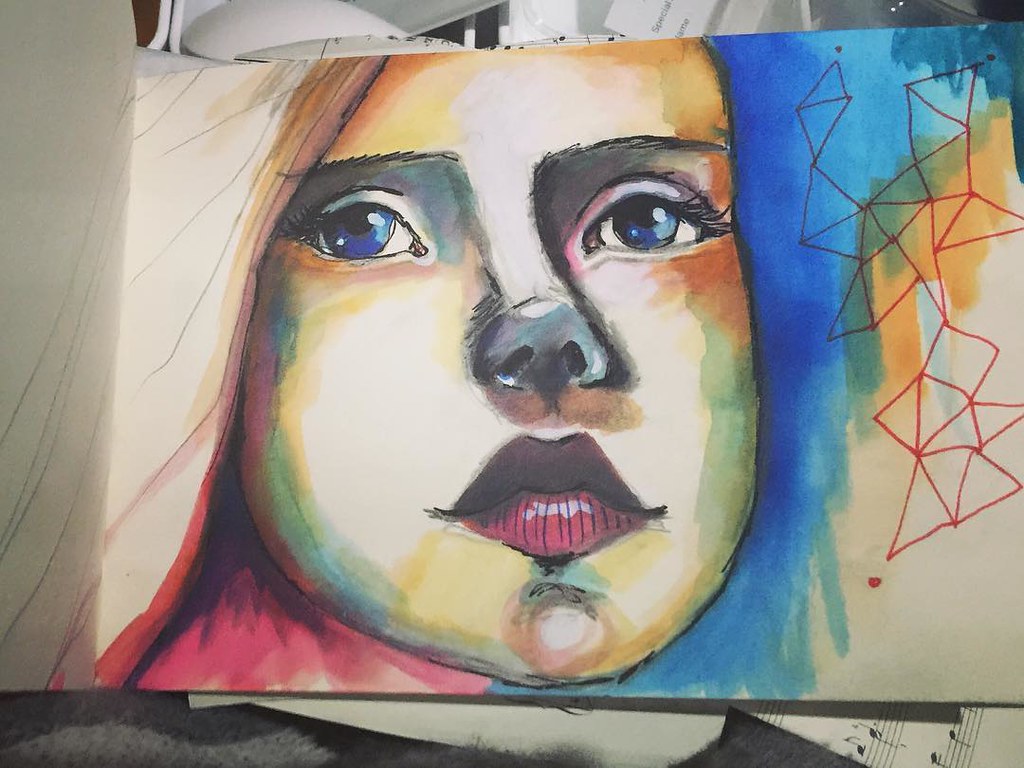This image showcases a photograph of a watercolor painting, likely created in a sketchbook as suggested by the visible spine on the left side. The artwork features a close-up portrait of a young girl with strikingly large, blue eyes, and red, slightly two-toned lips. Her simple, uncolored hair is positioned to the left of her face. The artwork incorporates abstract elements, including geometric designs on the right side of her face, which resemble origami patterns rendered in red ink. Surrounding these features, the artist has added random patches of blue and red coloration, emphasizing a blend of both abstract and minimalist styles.